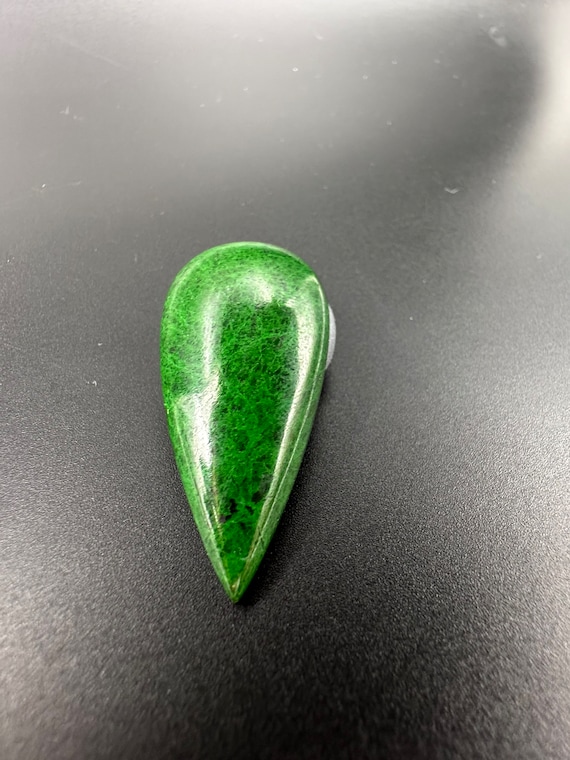This photograph features a vertically oriented, portrait layout with a background consisting of varying shades of black, charcoal, and light gray. The texture of the background appears slightly grainy, reminiscent of a plasticky surface with subtle light reflections, particularly along the top and right sides, creating areas of lighter gray where light, possibly sunlight, hits.

At the very center of the image lies an upside-down teardrop-shaped object, which looks like a striking emerald-green stone. The stone has a marbled texture, incorporating shades of darker green and black, with certain spots highlighted by white reflections due to the lighting. The shape of the stone starts with a rounded top, tapering down to a pointed end. There's an etched line running through its middle, hinting that it might be composed of two pieces joined together. The exact size of this intriguing green stone is indeterminable because there is no adjacent object for reference scale. Notably, there are no other objects, people, or text in the image, concentrating all visual interest on the solitary jewel-like stone against the understated background.